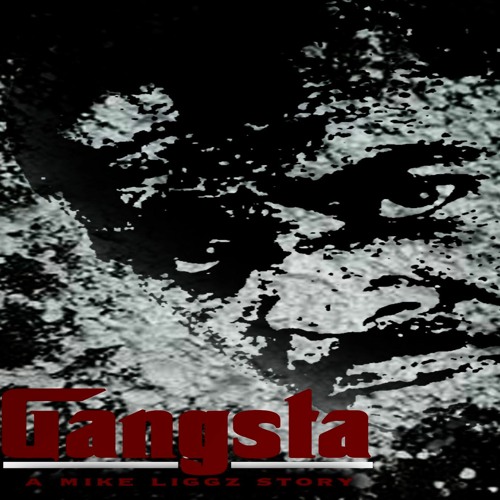The image is a striking, black-and-white piece that looks like it could serve as a poster, an album cover, or a book cover. Dominating the image is the black and gray outline of a stern-faced man with a mustache and goatee, his face rendered in a speckled, almost pointillist style that gives it a surreal, powdery texture. It's as if his visage is materializing through a mist of white powder insinuated to be cocaine, creating a haunting, abstract effect. The man's intense gaze is fixated outward, his head slightly tilted to the left while his eyes look to the right, giving a sense of deep contemplation or menace.

Across the bottom left of the image, bold red text spells out "Gangsta" in a stylized font reminiscent of The Godfather's iconic typography. This title is underlined by a thick white line, disrupted only by the "G" of "Gangsta." Beneath this title, also in red, is the subtitle "a Mike Liggs story," standing out against the darker tones of the background. The interplay of black, gray, and red, alongside the textured depiction of the face, imbues the image with a dramatic and gritty atmosphere, suggesting a gripping narrative tied to themes of danger and intense personal conflict.